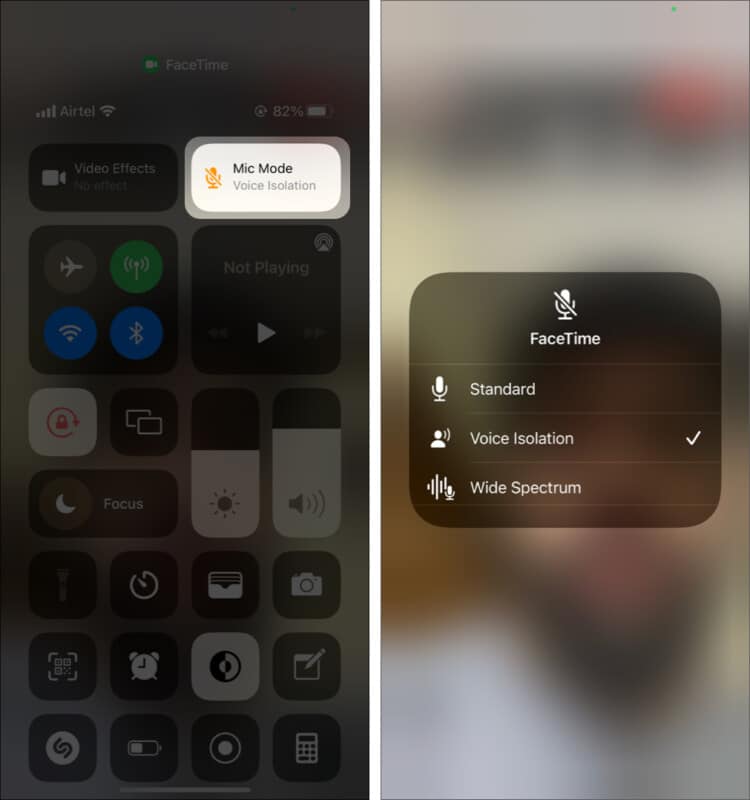The image on the website features a close-up of a smartphone screen. The primary focus is on an active FaceTime call interface. Due to the overall darkness of the photograph, details are somewhat obscured, giving the impression of a gray overlay. Notably, the FaceTime indicator is clearly visible at the top of the screen, accompanied by a faint green icon. The battery status is displayed at 82%, and the device shows a strong signal connection.

The main section of the screen prominently displays the "Mic Mode" options within the FaceTime app. The highlighted selection is "Voice Isolation," with other available options like "Standard" and "Wide Spectrum" also visible but less emphasized. Icons for various settings such as airplane mode, Wi-Fi, and media playback status ("Not Playing") are displayed in a black box with an arrow.

Additionally, the lower portion of the screen features various control icons, including those for adjusting volume and brightness. Among these, the "Focus" mode is noted, along with tiny icons for time and battery status.

On the side of the phone facing the camera, the image is quite blurred, but the FaceTime interface is again visible, featuring a microphone icon at the top. The "Voice Isolation" option is distinctly marked with a white check mark, indicating it is currently selected.